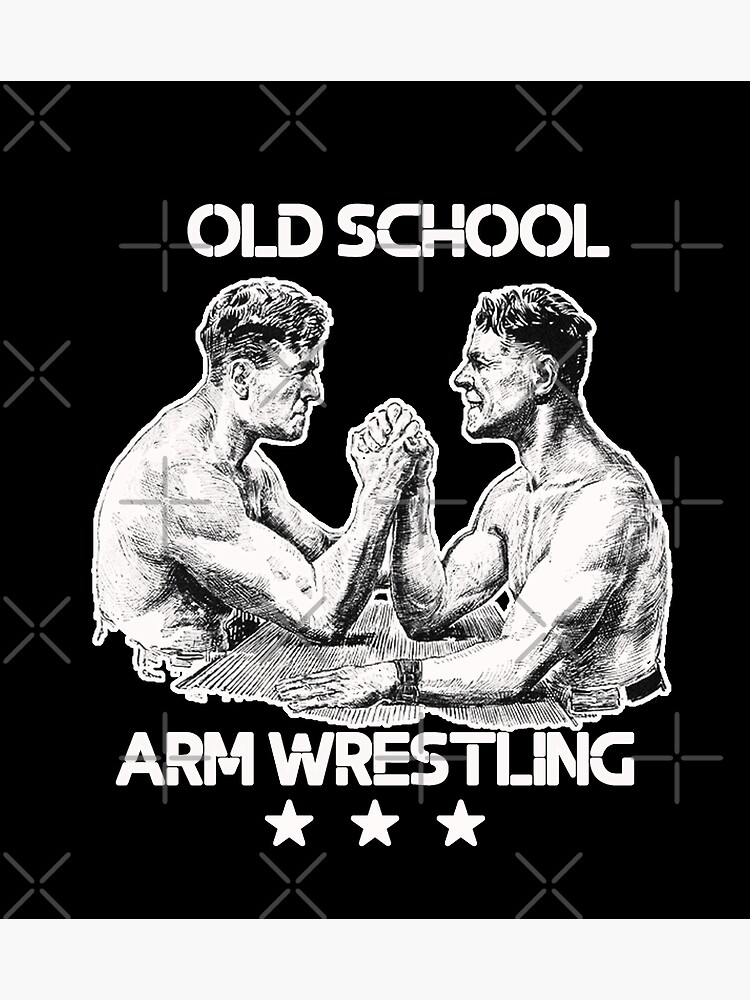The poster features a striking image centered on a perfect black square that serves as the backdrop, adorned with a pattern of alternating light gray X’s and plus signs. At the top of the black square, in bold white letters, the caption "OLD SCHOOL" stands prominently. Below this title, a compelling black-and-white sketch depicts two bare-chested gentlemen in the throes of an intense arm wrestling match. Their hands are tightly locked over a wooden table, with their free arms resting beside them; one individual notably wears a wristband or watch. Both men have short hair and determined expressions as they strain against one another. The table, rendered in a slightly surreal, folding manner, adds to the dynamic tension of the scene. Beneath the arm-wrestling image, the words "ARM WRESTLING" appear in the same bold white font, followed by a line of three solid white stars, completing the vintage and powerful design of the poster.